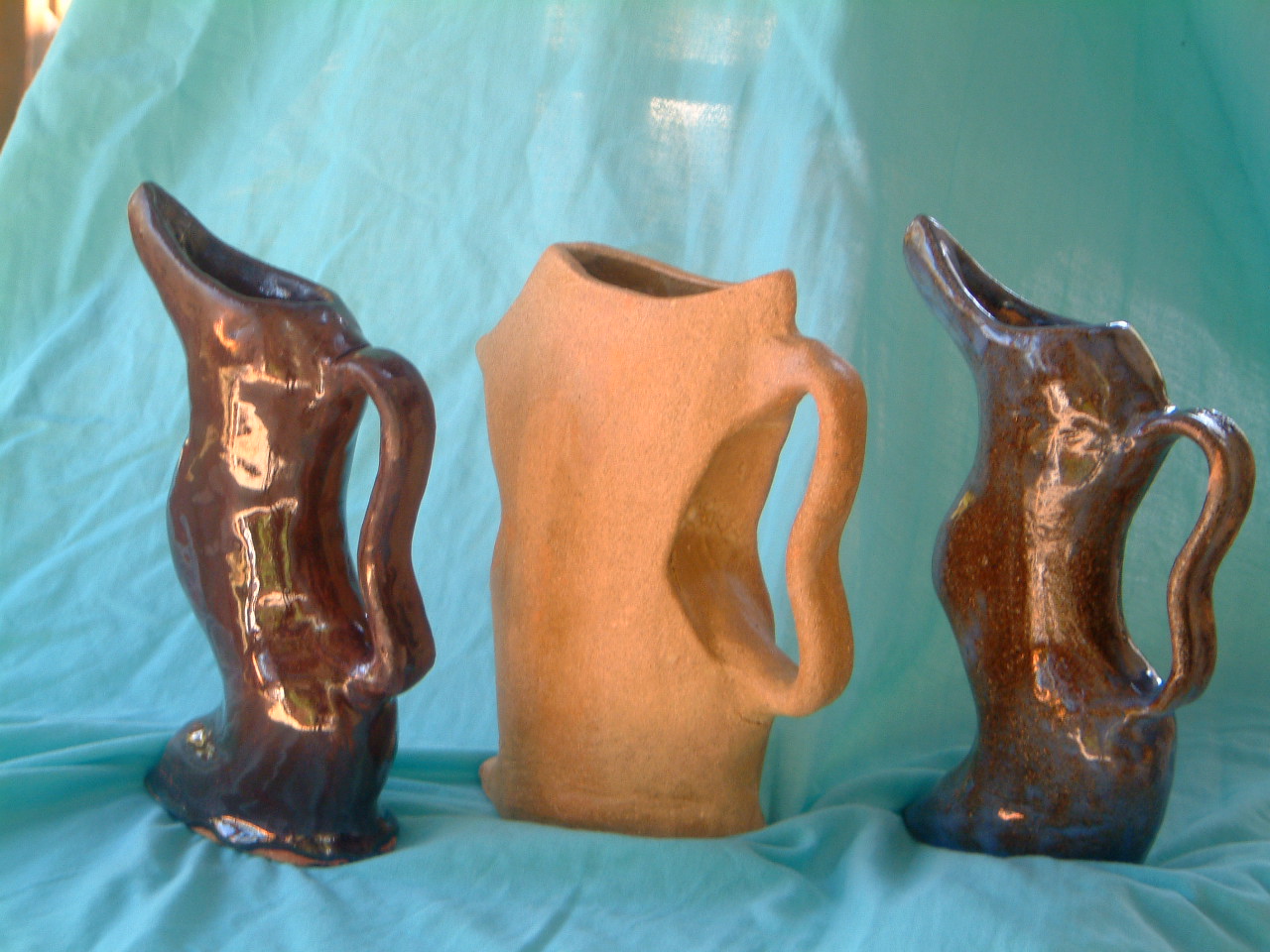The image features three ancient-looking pots arranged on a teal-colored sheet that flows and drapes beneath them. The two pots on either side are identical with a shimmering brown-bronze color, each featuring a curved handle and a beak-like spout on the left-hand side. These pots have a triangular shape and a reflective surface. In contrast, the middle pot is slightly wider and made of a matte, stone-like material in an orangish-beige hue, with a heart-shaped handle and a simple rounded opening at the top. All three pots are of different sizes and textures but share a similarly historical aesthetic.